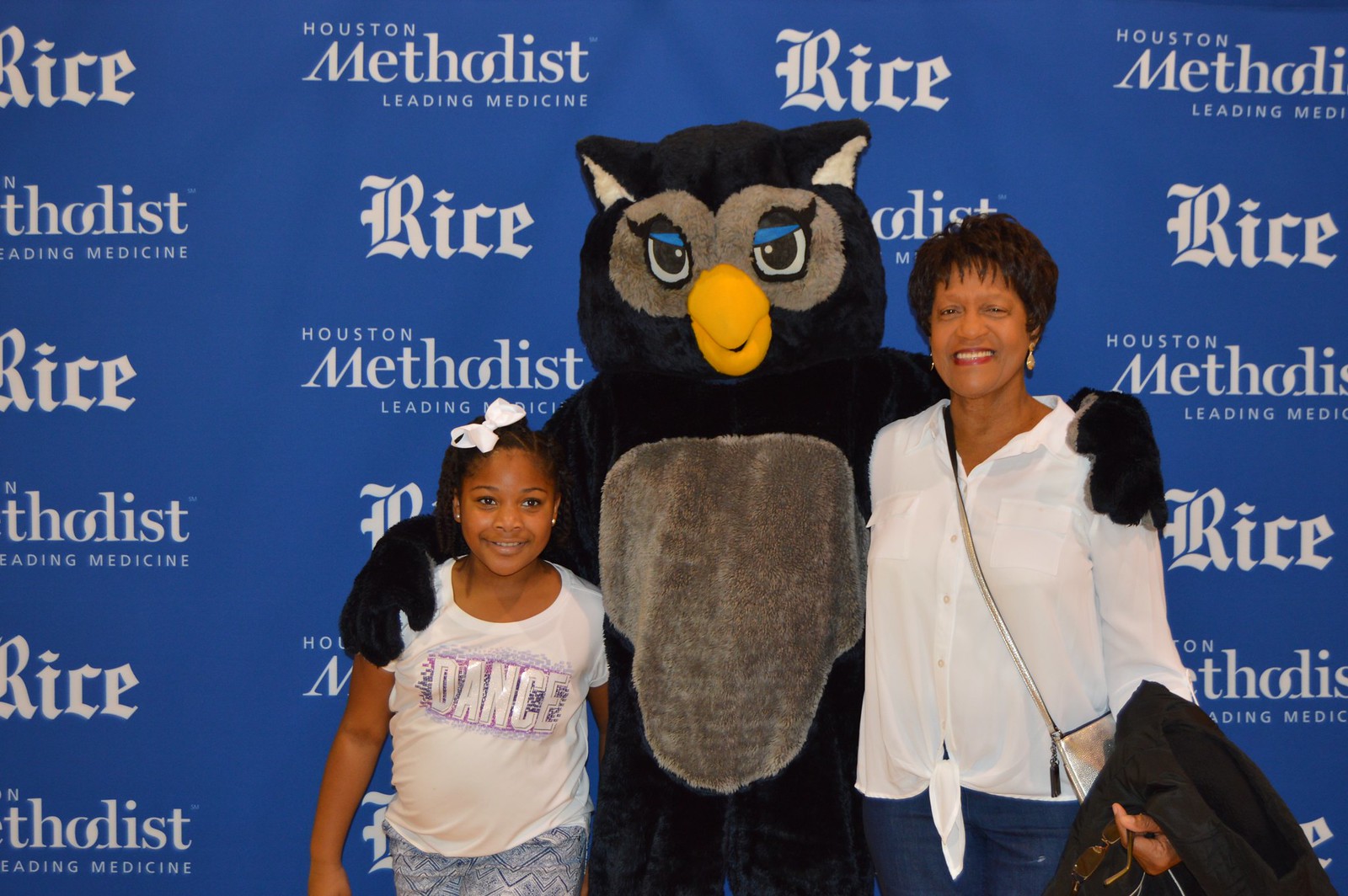In this image, a vibrant scene unfolds at a media day event. Posed in front of a blue backdrop adorned with the repeating words "Houston Methodist Leading Medicine" and "Rice University," three figures beam with joy. Central to the image is a whimsical owl mascot in a striking costume of blue with a gray belly, gray accents around the eyes, ear tufts, and a yellow beak. The owl has its wings draped affectionately over the shoulders of two individuals. On the owl’s left side stands a young black girl, her hair styled in braids adorned with a white bow. She wears a white t-shirt emblazoned with the word "Dance" and blue jeans. On the owl’s right side is an older woman with short hair, clad in a white blouse and blue jeans. She accessorizes with a silver purse slung over her left shoulder and holds a jacket and a pair of sunglasses in her hands. Both the girl and the woman wear delighted smiles, capturing the warm, celebratory atmosphere of the event.